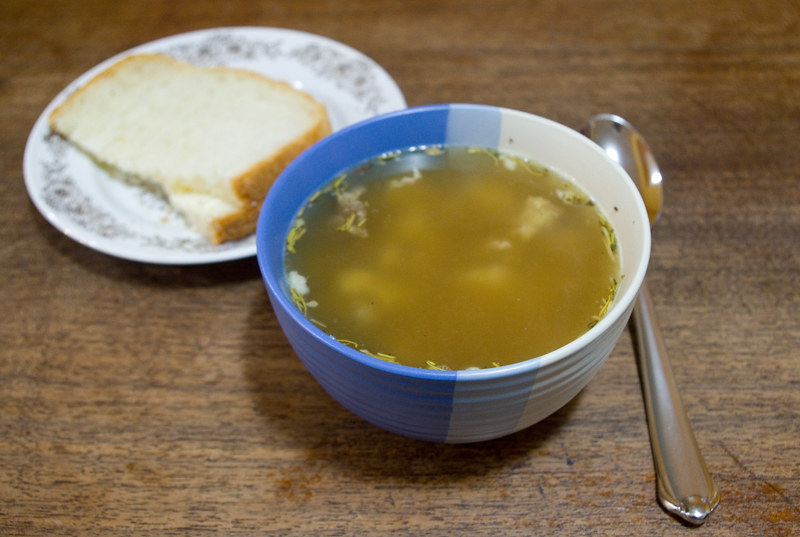In this photograph, a warm and inviting meal is captured from an elevated angle, showcasing a small bowl of soup and a plate with a sandwich, all set on a rustic wooden table. The soup features a cloudy, greenish-yellowish broth with visible pieces of food stuffs submerged within, possibly chicken and various spices, suggesting a hearty chicken noodle essence. The bowl itself is distinctive, with a blue gradient from darker on the left to lighter in the middle, transitioning to white on the right. A metal spoon rests to the right of the bowl, poised for use. Behind the bowl, slightly out of focus, sits a small, white plate with a decorative edge, holding a half sandwich made from what looks like two halves of a single piece of white bread. The composition thoughtfully emphasizes the textures and colors of the meal, creating a homely and appetizing scene.